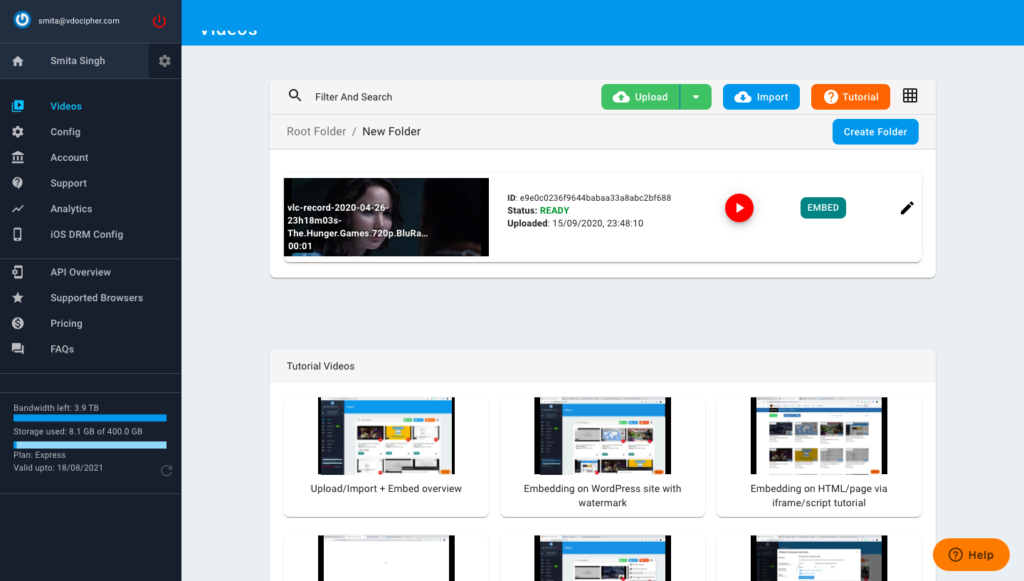Screenshot Description:

The screenshot captures a web page layout with distinct sections and elements. The page is divided vertically with a wide black border running down the left side. Adjacent to the black border, at the top of the page, is a blue horizontal banner stretching across the width of the screen. 

On the right side of the page, the background is gray, contrasting with two white rectangular boxes overlaid on this gray section. The top white box features options such as "Filter" and "Search Root Folder / New Folder," along with buttons labeled "Upload," "Import," "Tutorial," and "Create Folder." 

Below these controls, a thumbnail preview of a video displays an image of a woman with dark hair looking slightly to the right. Beneath this video thumbnail is another white box containing six smaller thumbnail photographs arranged in two rows: three on the top row and three on the bottom row. These thumbnails represent tutorial videos.

On the left-hand side, over the black border, a vertical list of text navigational links includes the following items: "Smita Singh," "Videos," "Config," "Accounts," "Support," "Analytics," "iOS," "DRM Config," "API Overview," "Supported Browsers," "Pricing," and "FAQs."

Overall, the page appears to be a user interface for managing and interacting with video content.